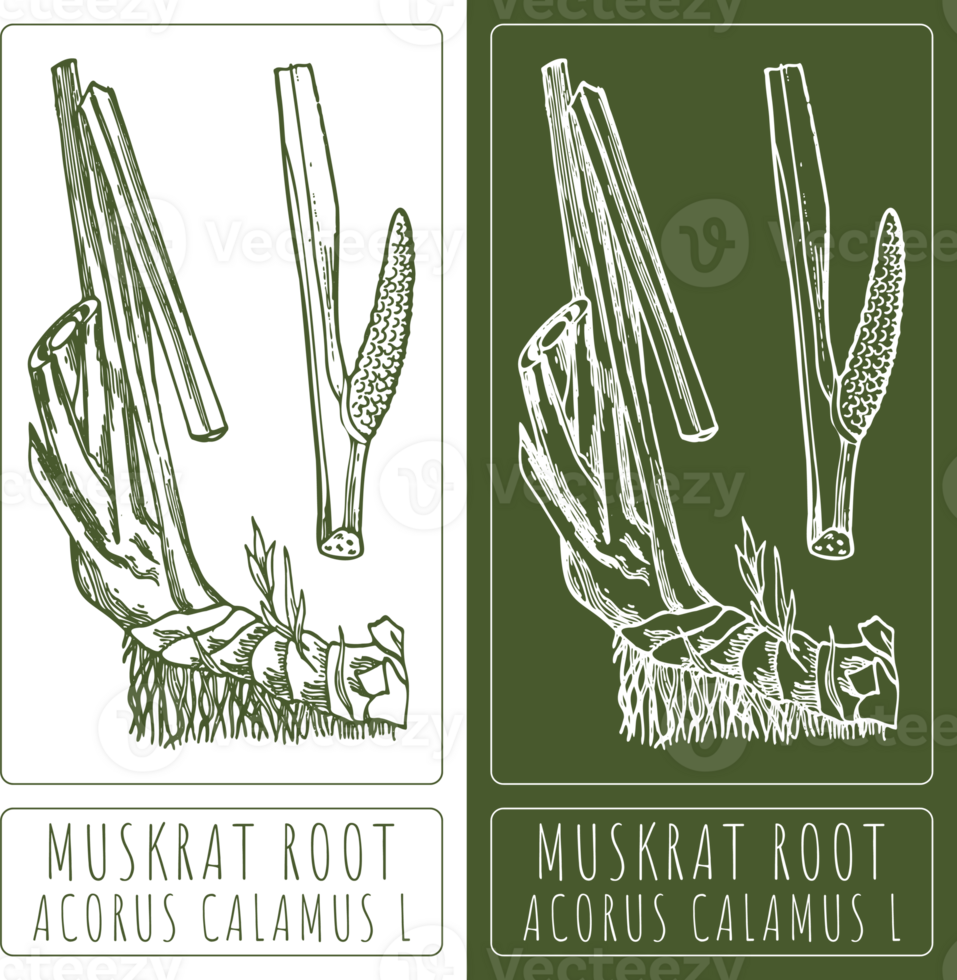The image features two vertically-oriented, side-by-side rectangular panels that are negative images of each other. The left panel has a white background with an olive green drawing, while the right panel features an olive green background with a white drawing. Both panels depict the same botanical illustration of "Muskrat Root, Acorus Calamus L.," which is labeled in all caps at the bottom in a thin line border. The left panel shows the text in green against the white background, and the right panel displays it in white against the green background. 

The illustrated plant appears as a cutting with small leaf shoots emerging, indicating signs of regrowth. The drawing includes an L-shaped piece on the left side and a Y-shaped piece on the right, with knobby, forked protrusions that might be seeds or flowers. The drawing shows the plant's roots extending downward. The olive green side has a pattern of watermarks featuring a logo with a "V" and the word "Vecteezy," distributed across the background. A thin line border also surrounds the plant illustration on each panel.